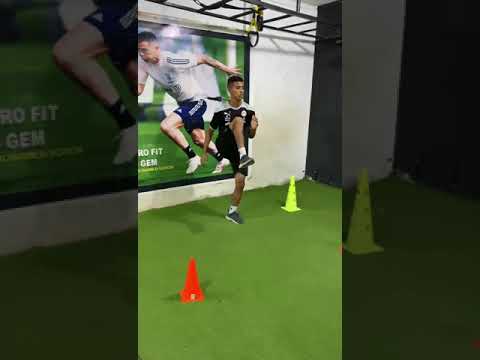The photograph is sectioned into three vertical panels, with the outer panels showing blurred, fragmentary parts of the central image. In the center third, a man in a black jersey with white shoulder accents, white socks, and gray sneakers with white soles practices soccer footwork. His right knee is raised high to his chest while his left leg is slightly lifted. He has brown skin and black hair. Behind him, a large, partially visible poster depicts a soccer player mid-run, wearing a white jersey, blue socks, and white shoes. The poster includes text fragments reading "RO...FIT" and "GEM." Parallel to the man’s body stands a yellow cone, and an orange cone lies diagonally down to his left, set on a surface of either astroturf or practice grass. The left and right thirds of the image obscure and repeat elements from the center, adding a layered, dynamic quality to the overall composition.